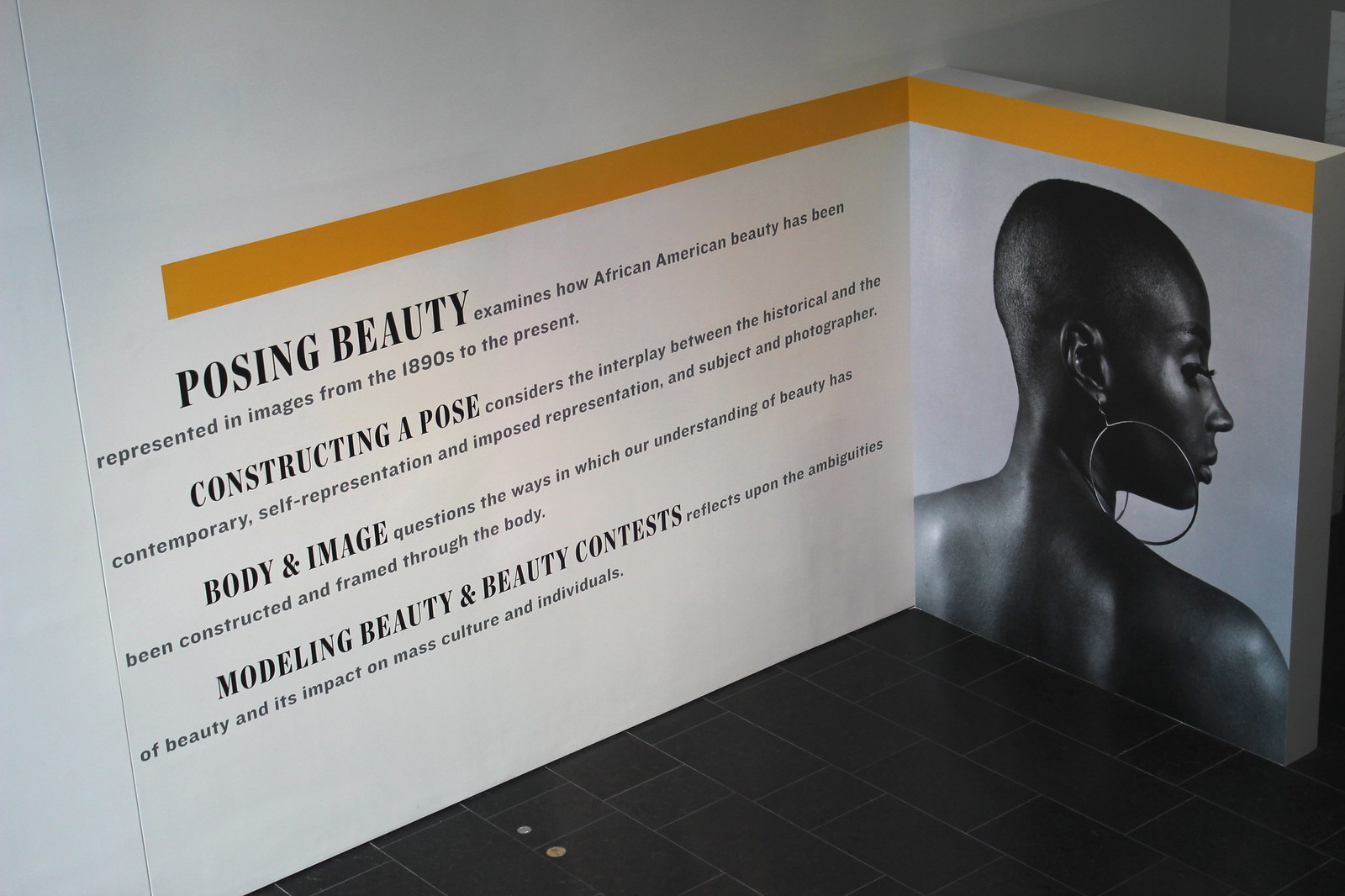This image captures an art exhibit display likely set in a museum. The scene is framed by a pristine white wall with an orange stripe along the top and a sleek black tile floor. Central to the visual narrative is a striking photograph of a black woman with closely shaved hair, dark and radiant skin, and adorned with a single large hoop earring. She is posed with her bare shoulders and neck visible, her body turned away but her head turned slightly to the right, offering a serene profile.

The text on the wall beneath the orange stripe is prominent and educational. In bold letters, it introduces the exhibit as "Posing Beauty," which examines the portrayal of African-American beauty in images from the 1890s to the present. Subsequent sections of text in varying font sizes elaborate on specific themes: "Constructing a Pose" delves into the interplay of historical and contemporary self-representation in photography; "Body and Image" questions the construction and framing of beauty through the physical form; and "Modeling Beauty and Beauty Contests" reflects on the complexities of beauty and its cultural and individual impacts. The woman's image, paired with the illuminating text, forms a cohesive and thought-provoking presentation on aesthetics and representation.